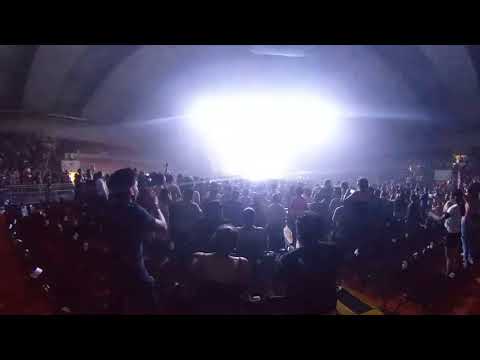The image depicts a massive indoor event, possibly a concert or large gathering, held in a building or stadium with a prominent arched concrete ceiling. The venue features a domed roof and is filled with thousands of people of all ages—men, women, and children—who are predominantly seated in regular chairs on the ground level, while additional stands are visible on the left and right sides. The entire crowd faces towards a stage, which is illuminated by intense, bright white lights that obscure any activity on it, making it difficult to discern specific details of the performance or event. The colors prevalent in the scene include black, gray, white, light blue, red, tan, and yellow. The setting clearly indicates an indoor concert venue filled with vibrant energy, with intricate architectural elements like balconies or upper-level stands contributing to the grandeur of the space.